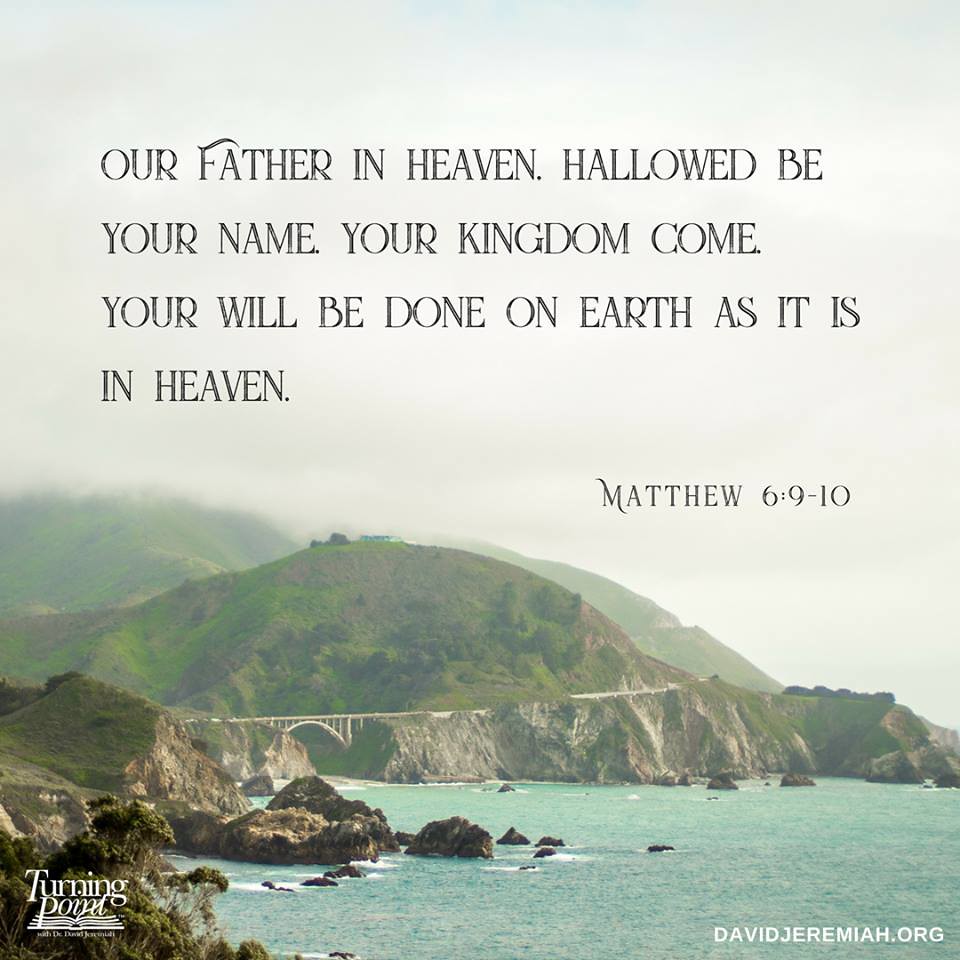The image features a scenic view of California's Highway 1 and the iconic Bixby Bridge, captured from a distance on a cloudy day with a marine layer and fog hovering over the green, tree-dotted mountains. The upper half of the image is dominated by the cloudy, white sky, with an inspirational quote from the Bible in large black capital letters: "Our Father in heaven, hallowed be Your name. Your kingdom come, Your will be done on earth as it is in heaven." (Matthew 6:9-10). The quote is arranged on four lines, prominently displayed against the sky. The lower right corner of the image, in white text, features the website davidjeremiah.org, while the lower left corner displays the logo of the organization "Turning Point," an illustration resembling a book laid flat. The scene below the quote includes rolling green hills, rocky areas extending into a deep blue body of water, and a few scattered trees, creating a serene and picturesque setting.